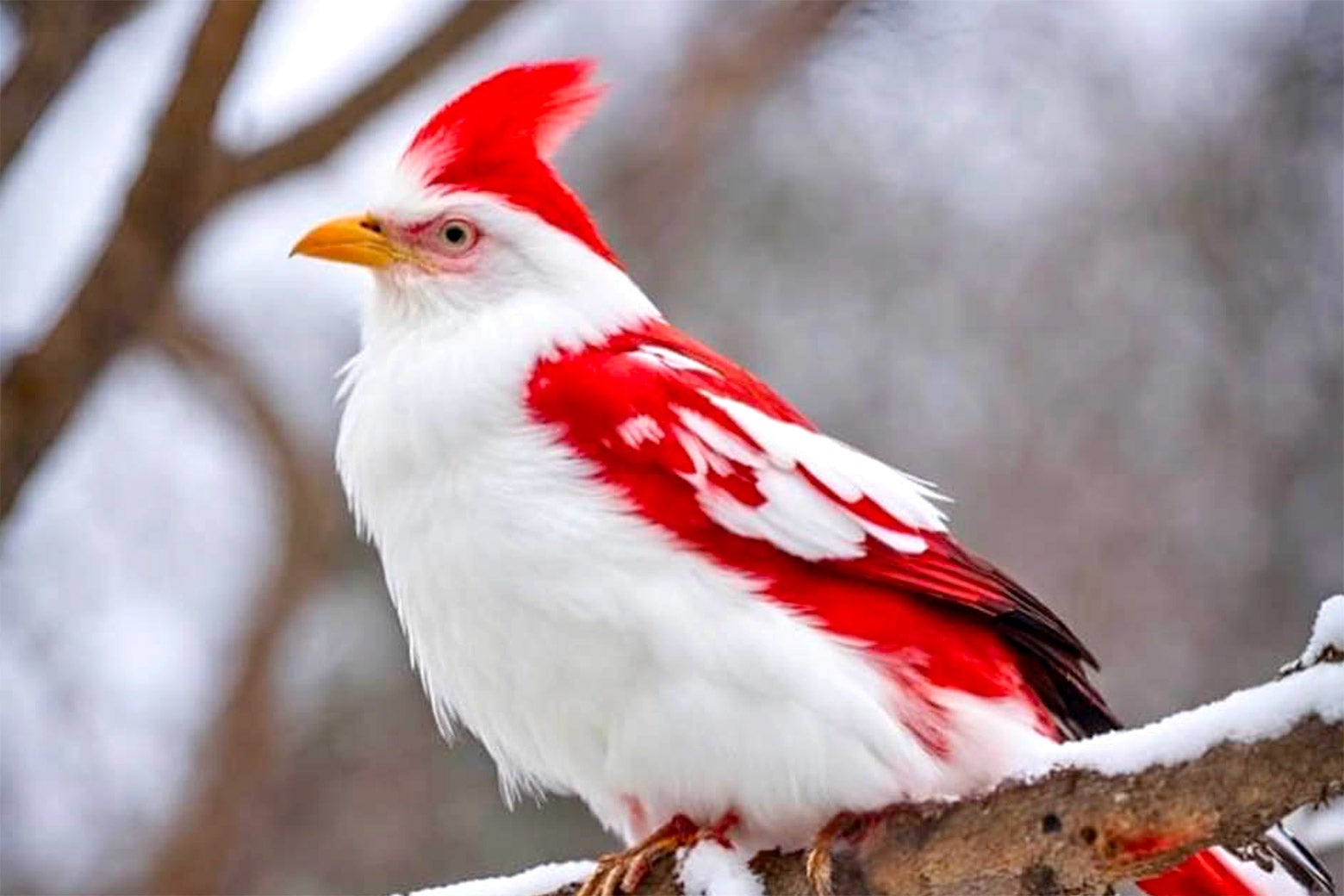In this close-up photograph, a bird with a striking yellow beak is the central focus. The bird is perched on a snow-covered tree branch, surrounded by an out-of-focus woodland area devoid of leaves, suggesting a cold winter day. The bird’s plumage displays a vivid combination of colors: its head and underbelly are white, its eyes are black, and it sports a distinctive red fin-like crest atop its head. Its wings are a beautiful blend of red feathers with white accents and black tips, while its feet are brown. The overall setting creates a serene and chilly atmosphere, with the bird standing out against the muted, blurred backdrop.